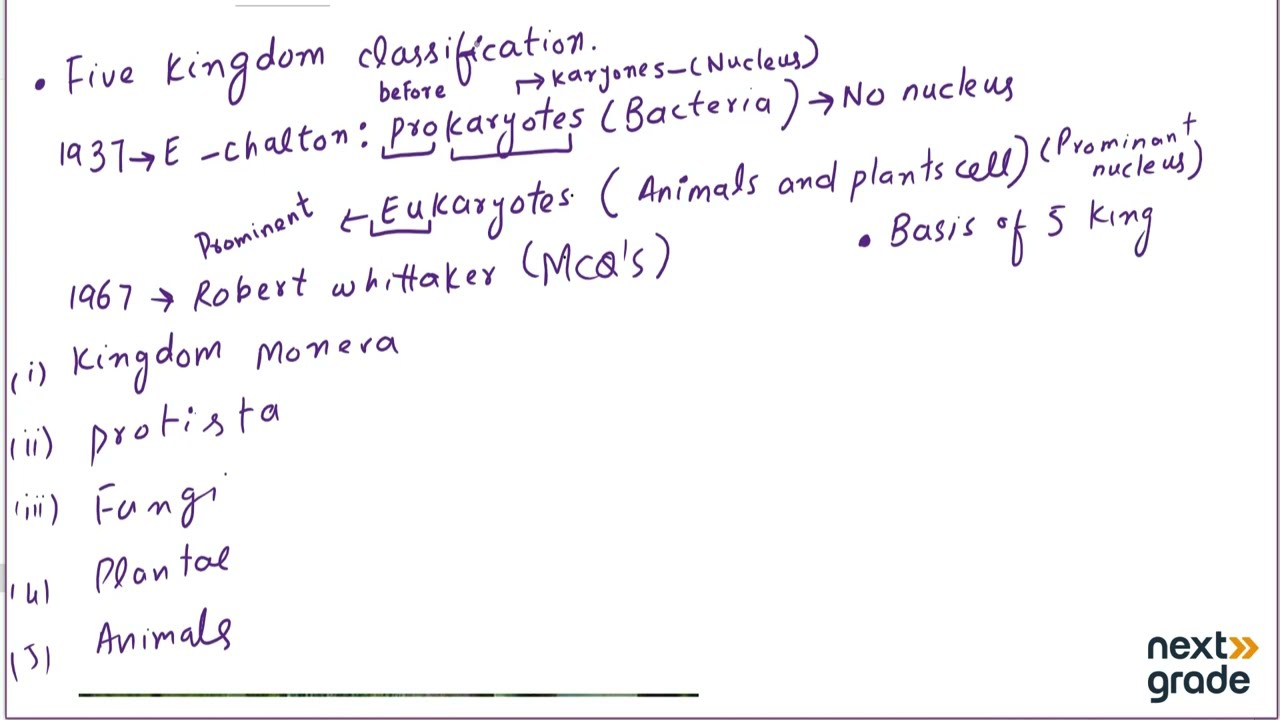This image showcases neatly handwritten notes set against a solid white background, appearing to be created digitally, likely on an iPad. The notes, written in a blackish-purplish font, delve into the five kingdom classification system from a biology class. The top of the document prominently features the title "Five Kingdom Classification" next to a bullet point, indicating the structure and topics covered. Important historical dates such as 1937 and 1967 are mentioned, aligning with significant contributions, including Robert Whittaker's work, to the understanding of prokaryotes and eukaryotes. Detailed classification follows with five clearly numbered kingdoms: Monera, Protista, Fungi, Plantae, and Animals. These notes provide definitions and characteristics, including specifics like "prokaryotes" and "no nucleus" under bacteria. The document is thorough and well-organized, making complex biological concepts accessible. In the bottom right corner, the logo "Next Grade," accented with two yellow arrows, is prominently displayed, signifying the potential educational tool or platform used to create these notes.